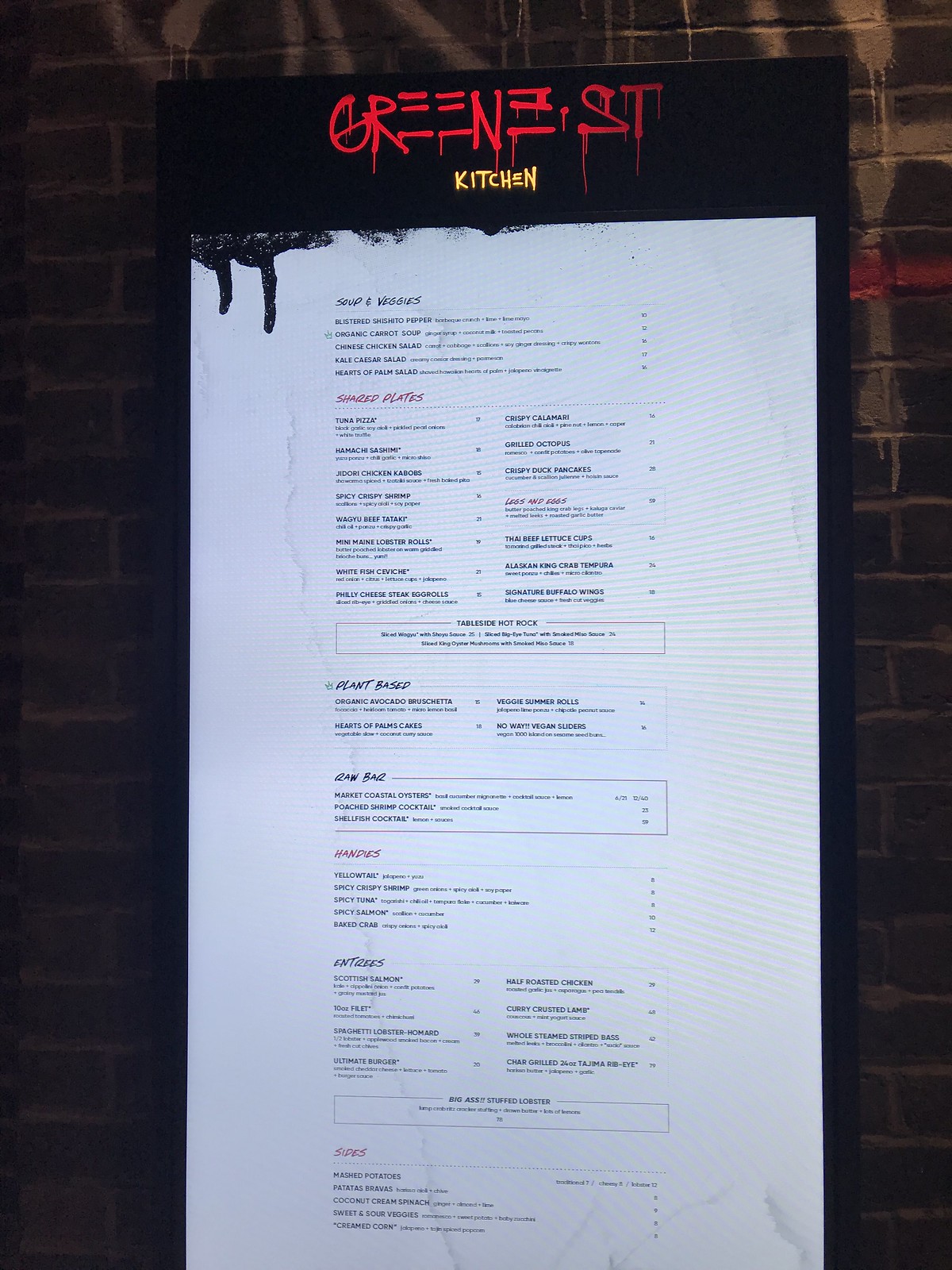The photograph showcases the menu for Green Street Kitchen, prominently displayed on a nearly black brick surface that adds a sophisticated backdrop. At the very top of the menu, the restaurant's name, "GREEN STREET KITCHEN," is emblazoned in striking red letters. The menu itself is a pristine white paper encased in dark borders, creating a stark contrast.

Beneath the title, the menu begins with a section labeled "Soup and Veggies," followed by a list of items that are difficult to discern due to the small size of the photograph. Further down, a bold red heading reads "Shared Plates," under which several tempting dishes are listed, including "Crispy Calamari," "Grilled Octopus," "Crispy Duck Pancakes," and "Alaska King Crab Tempura." 

Toward the bottom, the menu highlights a section dedicated to "Plant-Based" meals, though some items in this category are partially obscured and hard to read. Another red heading, which appears to be "Hand," introduces selections like "Yellowtail" among others. 

The intricate details and diverse offerings of the menu hint at an eclectic dining experience, combining traditional and innovative culinary creations.